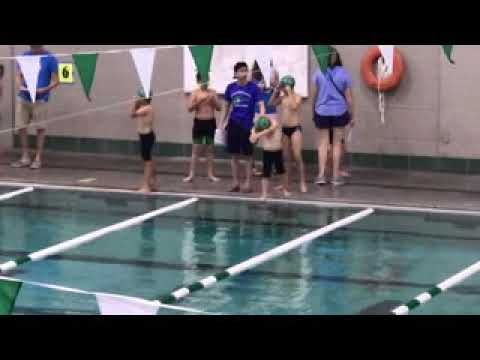The image captures an indoor swimming pool scene featuring four young boys, likely aged eight to nine, who appear to be either at a swim lesson or a tournament. The children are dressed uniformly in black swim trunks; three in shorts and one in speedos, all topped with green swim caps. They are positioned near the top center of the image, seemingly poised to dive into the clear blue water, sectioned off by white lane barriers.

In the foreground, a young man, probably their swim instructor, stands centrally with two children on either side. He is attired in a navy blue t-shirt with white lettering, black basketball shorts, and a black hat. To the left side, another adult partially visible, wears a dark blue top and light grey shorts. In the background, a woman in a lavender t-shirt, black shorts, and grey sneakers examines a chart on the wall, possibly indicating schedules or swim times. 

Additional elements in the image include a life preserver hanging on the wall in the upper right corner and a flag banner draped along the top, with parts hanging in the upper left corner. The pool's blue-tiled floor has a dark blue line running down the length, enhancing the organized, competitive atmosphere, while the number '6' is also visible on the wall, possibly marking a specific lane or section of the pool.